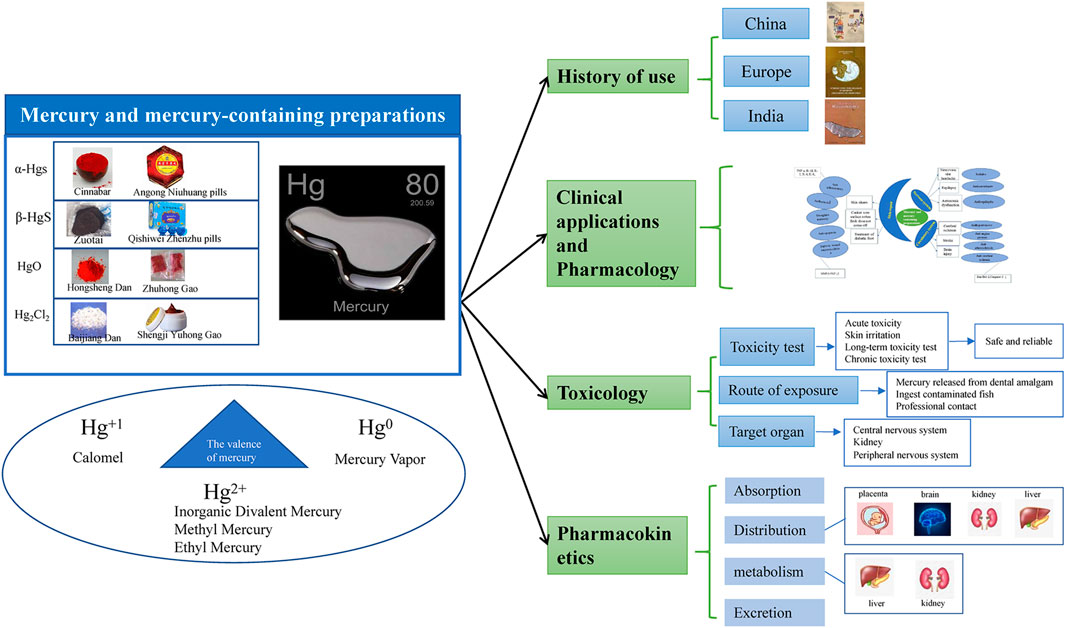This is a detailed horizontal chart focusing on mercury and mercury-containing preparations, featuring distinct sections linked by arrows. The left side starts with a blue-topped rectangle labeled "Mercury and Mercury-Containing Preparations," though the items listed underneath are unreadable. Adjacent, an oval with a blue triangle contains terms like calomel, mercury vapor, and different forms of mercury including inorganic divalent mercury, methylmercury, and ethylmercury, symbolized Hg2+. This section illustrates the balance of mercury. On the right, arrows extend from the initial blue rectangle to various green boxes that are titled "History of Use," “Clinical Application of Pharmacology,” “Toxicology,” and "Pharmacokinetics." The "History of Use" section lists regions like China, Europe, and India. The "Toxicology" box details toxicity tests, routes of exposure, and target organs, while "Pharmacokinetics" includes absorption, distribution, metabolism, and excretion processes. This complex diagram appears to serve educational purposes, possibly in pharmacology, illustrating the multifaceted use and effects of mercury.